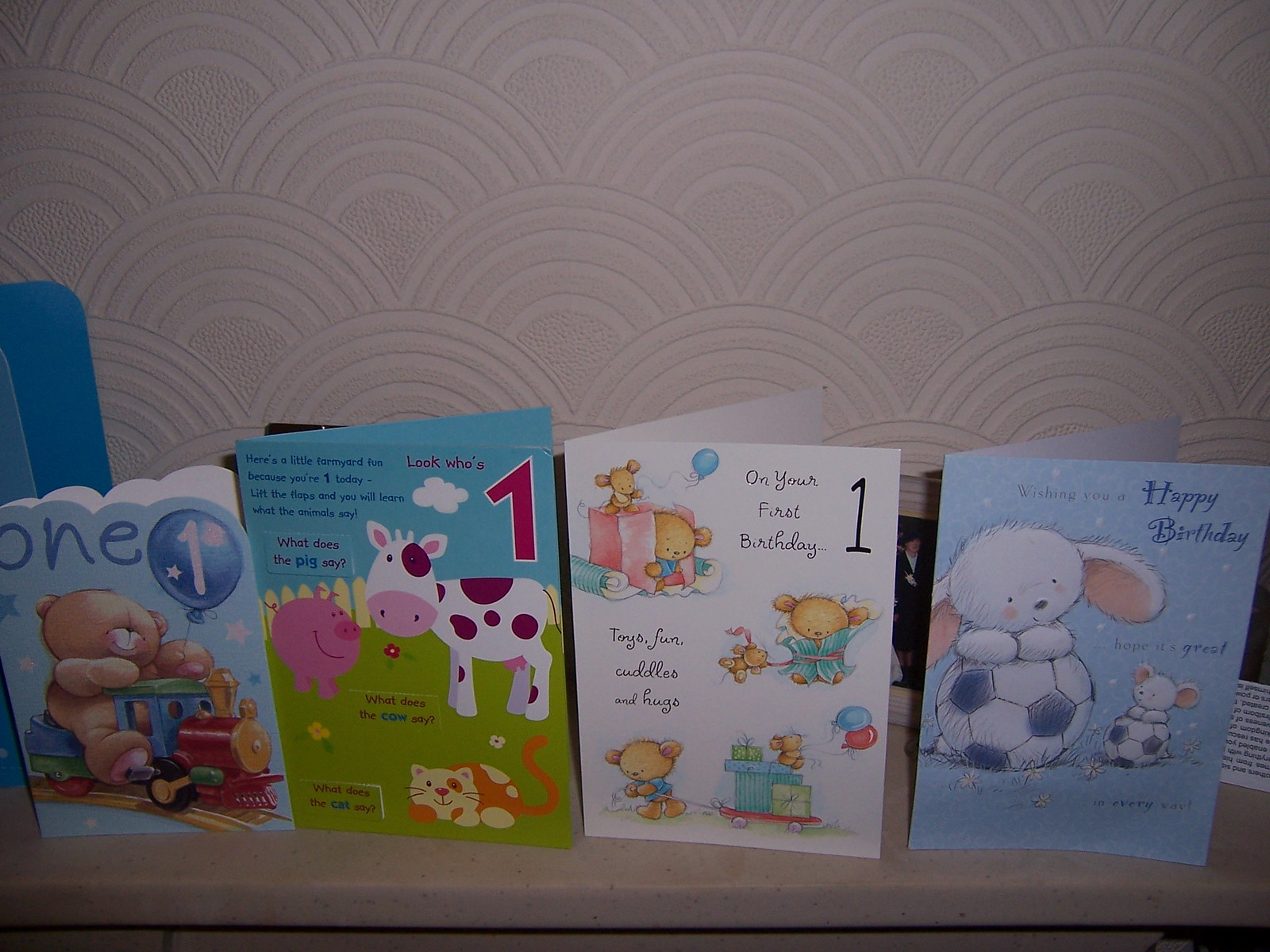This photograph features four vibrant and charming birthday cards, all propped up and standing upright on a table or shelf against a textured wall that resembles repeating hills or sunshine. Each card celebrates a child's first birthday. 

On the far left, the first card showcases a cheerful scene with a teddy bear riding a colorful train beneath a festive balloon, with the number "one" prominently displayed. Next, a playful card captures attention with farm animals—a cow, a pig, and a cat—accompanied by whimsical text like "look who's one" and fun phrases asking what each animal says. The third card, predominantly white, depicts adorable teddy bears surrounded by balloons and is inscribed with an endearing message: "on your first birthday, toys, fun, cuddles, and hugs." Finally, the fourth card features a delightful blue backdrop, where a white bunny, leaning over a soccer ball, extends "happy birthday" wishes and hopes for a day great in every way.

These cards, full of color and celebratory spirit, sit warmly against the textured background, evoking a sense of joyful festivity for a milestone first birthday.